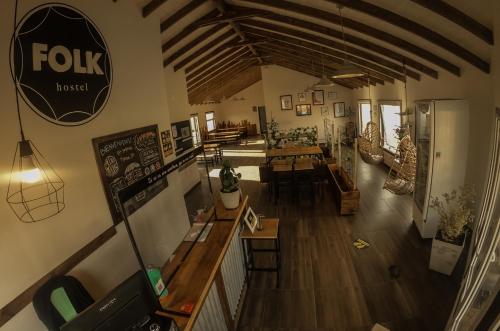This indoor photograph, seemingly captured from a high vantage point, likely a security camera, shows a cozy interior of what appears to be a small restaurant or bar with illuminated white and off-white yellow walls and rich wooden flooring. On the far left, a charming bar area features a sign that reads "Folk Hostel" in white lettering within a blue circle, accompanied by a chalk-drawn menu beneath it. This area is equipped with a glass counter where patrons can slip in their payments. Below this, towards the front of the image, a wooden counter adorned with plants, papers, and computers extends from the lower left-hand corner. Additionally, a single hanging light bulb is suspended by a wire, providing a dim light to the scene.

To the right of the bar, a series of wooden tables and benches are arranged comfortably in the background, hinting at the convivial atmosphere of the establishment. Framed pictures adorn the far wall on the left. The ceiling boasts natural dark wood beams, enhancing the rustic charm, while hanging lights add to the ambiance.

Towards the right side of the image are several windows allowing ample sunlight to pour in, casting light on the wooden floor and creating a warm, inviting glow. Next to these windows, innovative egg-shaped chairs hang from the ceiling, adding a unique design element. An antique fridge with a glass front stands on the right beside a potted plant, further contributing to the eclectic and homey feel of the space. The setting outside the windows is white and sunny, enhancing the overall brightness of this intimate dining area.